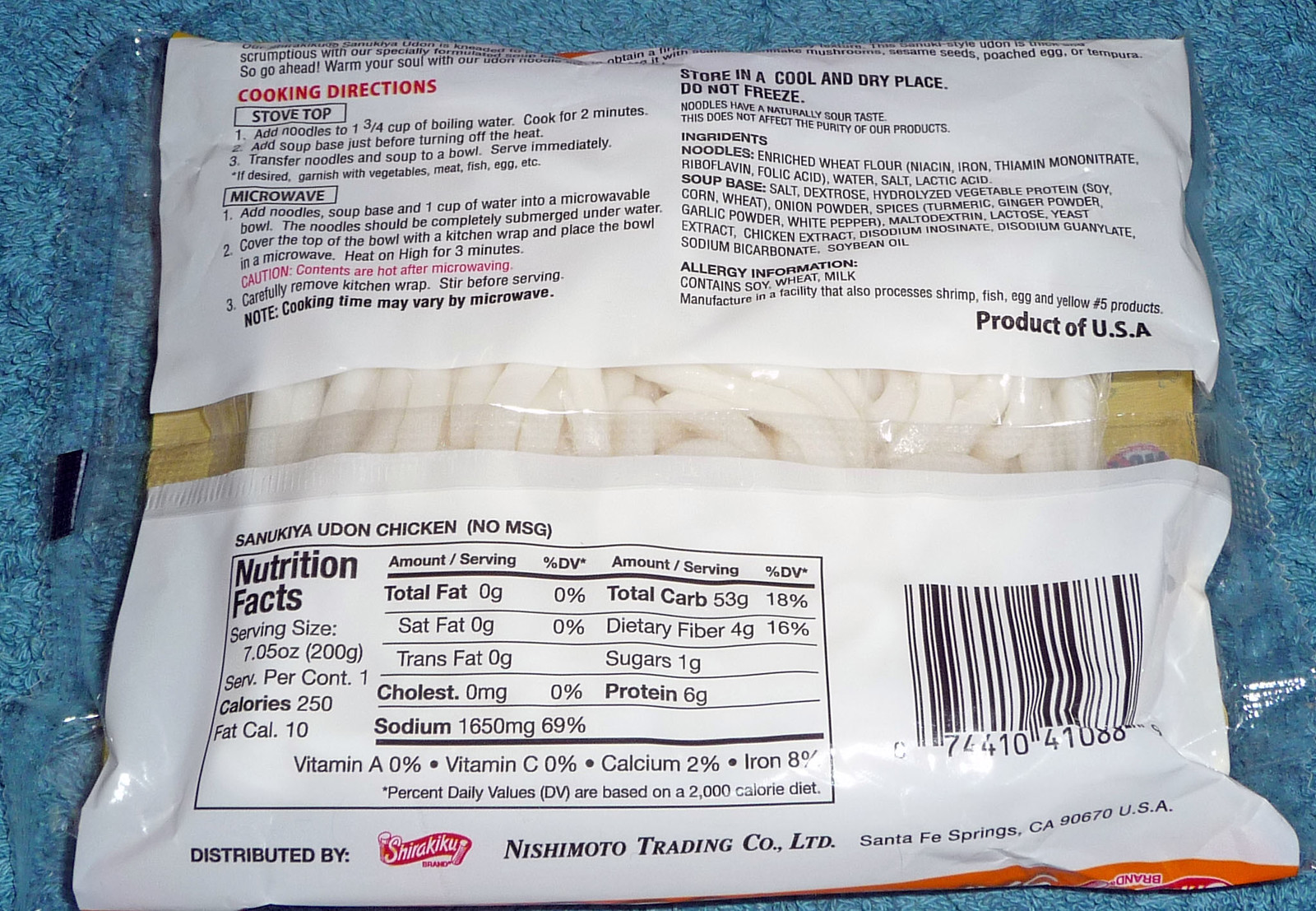On top of a blue granite or perhaps wooden table, there is a packaged food item whose details are clear on the labeling. The package prominently displays the nutrition facts, including cooking directions for both stovetop and microwave methods. The serving size is specified as 7.05 ounces (200 grams), with one serving per container. The package details that the total caloric content is 250, with 10 of those calories deriving from fat. Notably, the product is distributed by Nishimoto Trading Company Co. Ltd., clearly spelled out as N-I-S-H-I-M-O-T-O.